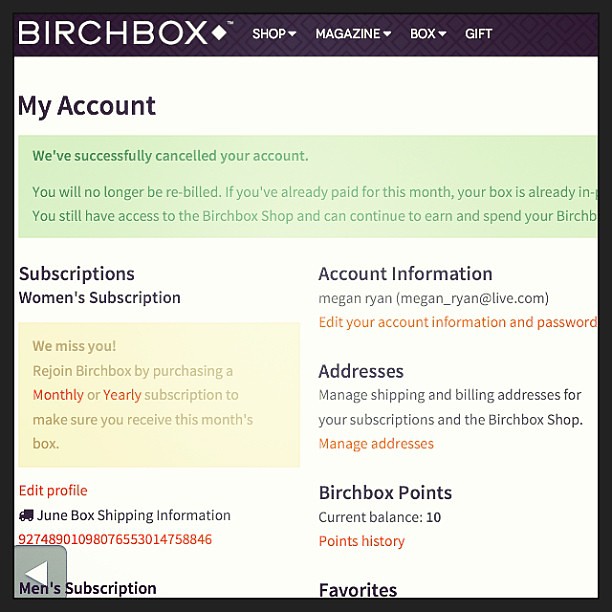This is a detailed screenshot of an account view on the Birchbox website. At the top, a dark banner features the Birchbox logo on the left, alongside navigation options for "Shop," "Magazine," "Box," and "Gift." Below the logo, the page title "My Account" is prominently displayed. A green notification box beneath the title declares, "We've Successfully Cancelled Your Account," indicating that the user will no longer be rebilled. There's also a message confirming that any payments made for the current month will still result in receiving this month's box.

Further down, the page is divided into multiple sections, including "Subscriptions," "Account Information," "Addresses," "Birchbox Points," and "Favorites." Under "Subscriptions," it specifies a "Women's Subscription" and provides the shipping information for the June box. There's also a small yellow box prompting the user to "Rejoin Birchbox by Purchasing a Monthly or Yearly Subscription to Make Sure You Receive This Month's Box."

The account owner's name is displayed as Megan Ryan, and she currently has a Birchbox points balance of 10, with an option to view her points history. The text at the bottom mentions that Megan will still have access to the Birchbox shop and can continue to earn and send Birchbox points.